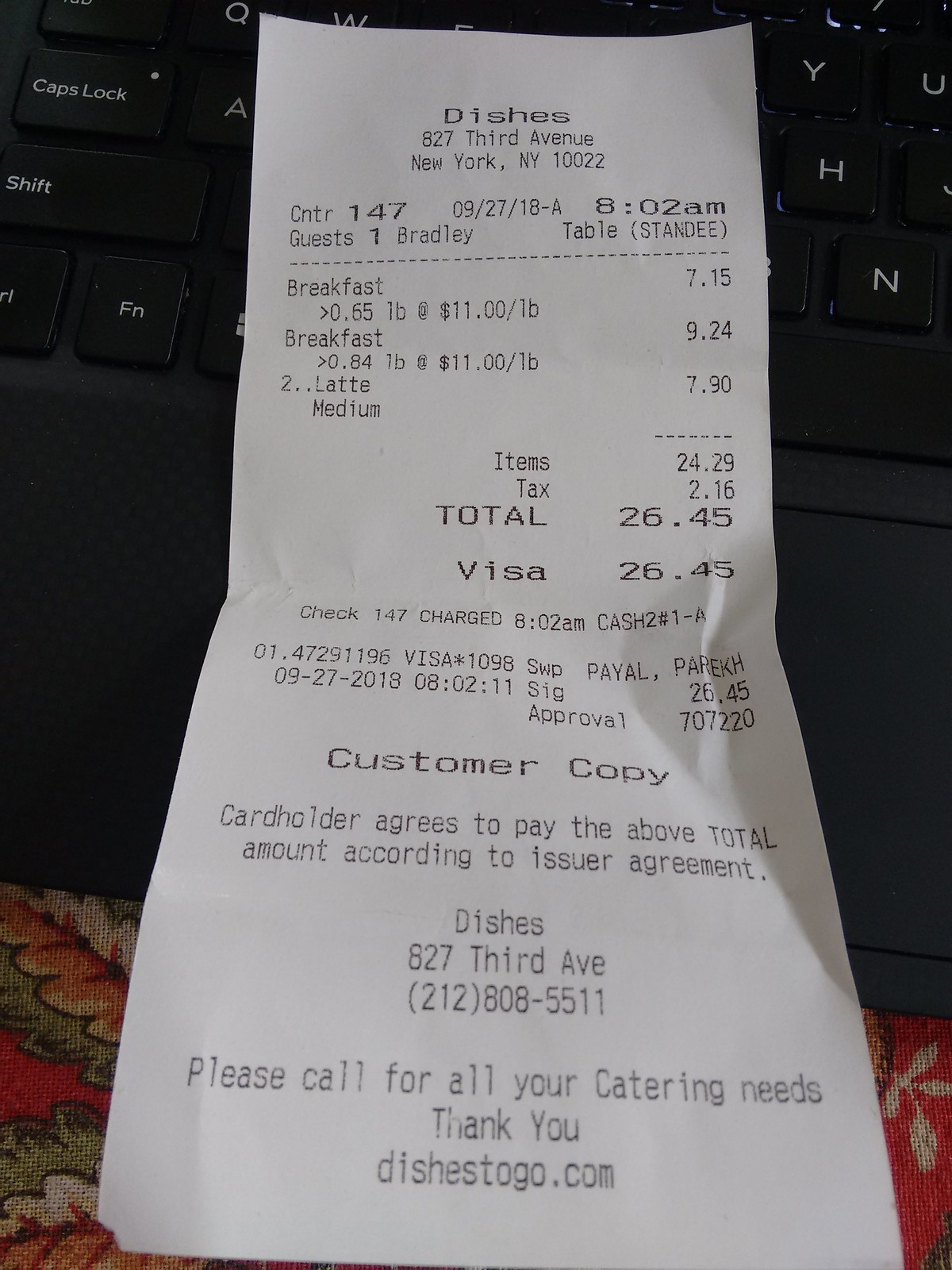This photograph captures a receipt placed on a standard QWERTY keyboard. The keyboard rests on an orange tablecloth adorned with green leaf prints. The receipt details a transaction from "Dishes," located at 827 3rd Avenue, New York, NY 10022. The time stamp reads 8:02 a.m., indicating service for one guest. The guest, named Bradley, ordered breakfast items including a $7.15 option, another breakfast item for $9.24, and two lattes costing $7.90. The subtotal of these items amounts to $24.29. With the addition of $2.16 in tax, the grand total comes to $26.45. The receipt also notes that the $26.45 payment was processed via Visa and includes the customer's copy.